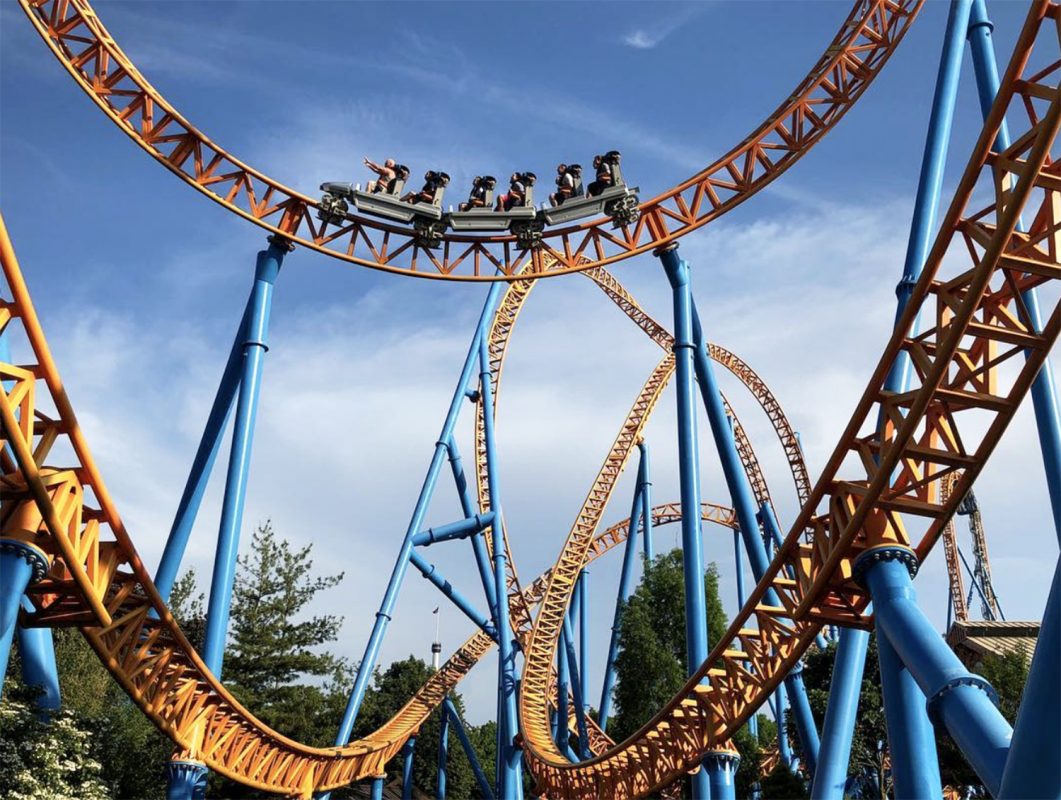The photo captures a dramatic, upward view of a sprawling roller coaster with a bright blue sky adorned with white clouds in the background. The roller coaster, characterized by its intricate, metallic framework, features a striking light orange track complemented by blue support columns. A single train with three cars, filled with 12 riders, ascends along the track. Each car, painted gray, seats two people per row in a paired configuration. The roller coaster twists and loops in a series of swoops and swirls, creating a thrilling visual spectacle. Lush green trees punctuate the lower part of the image, framing the towering amusement ride.